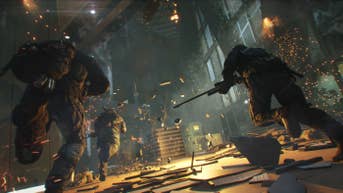In this dynamic scene captured from an animated cartoon or video game, we find ourselves in a vast indoor space with an industrial ambiance characterized by its high ceilings and large windows along one wall. The area is engulfed in chaos, with three military men in full combat gear sprinting forward, their faces a mix of determination and urgency. Each soldier wields a gun, prepared for whatever assault lies ahead. Around them, explosions erupt violently, sending showers of debris flying through the air. Sparks can be seen scattering in all directions, indicating they are under heavy enemy fire. The ground is littered with rubble, adding to the intensity and peril of their environment. The scene is a vivid portrayal of action and danger, highlighting the soldiers' bravery amidst the havoc.